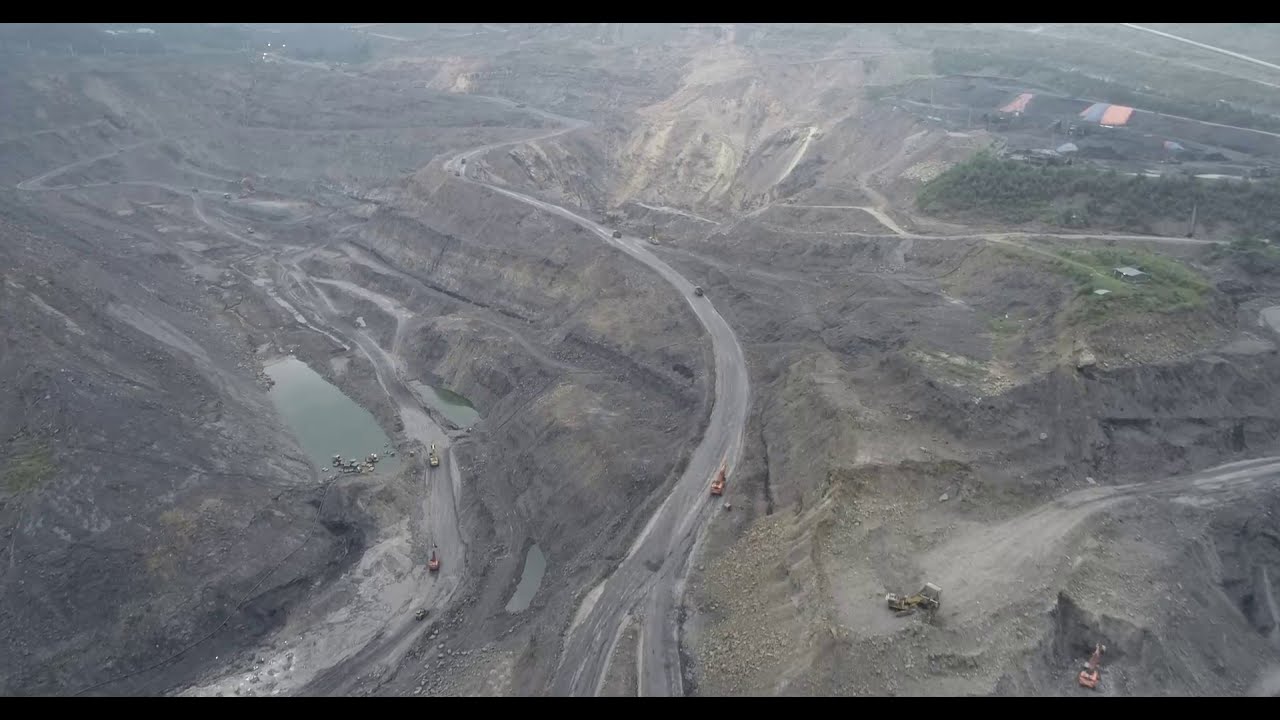This is an overhead, aerial shot of a vast, rocky mountainous area reminiscent of the Grand Canyon, captured in color and presented using photographic realism. The landscape is in a landscape orientation and inset into a slightly larger black background, forming narrow black strips at the top and bottom. Dominating the image is a long, winding road that meanders through the rugged terrain, with three vehicles navigating the twists and turns of this central driveway. On the left-hand side of the image, a large quarry pit filled with water is visible, resembling a small lake. The right side features a collection of construction vehicles, including yellow, brown, and red tractors, indicating ongoing excavation or construction activities. Sandy cliffs and eroded hillsides add to the rugged topography, while the background reveals large commercial buildings, possibly warehouses, one with a red roof and another with a blue roof. The overall atmosphere evokes the arid, canyon-like environments typical of desert regions, captured meticulously through drone photography.